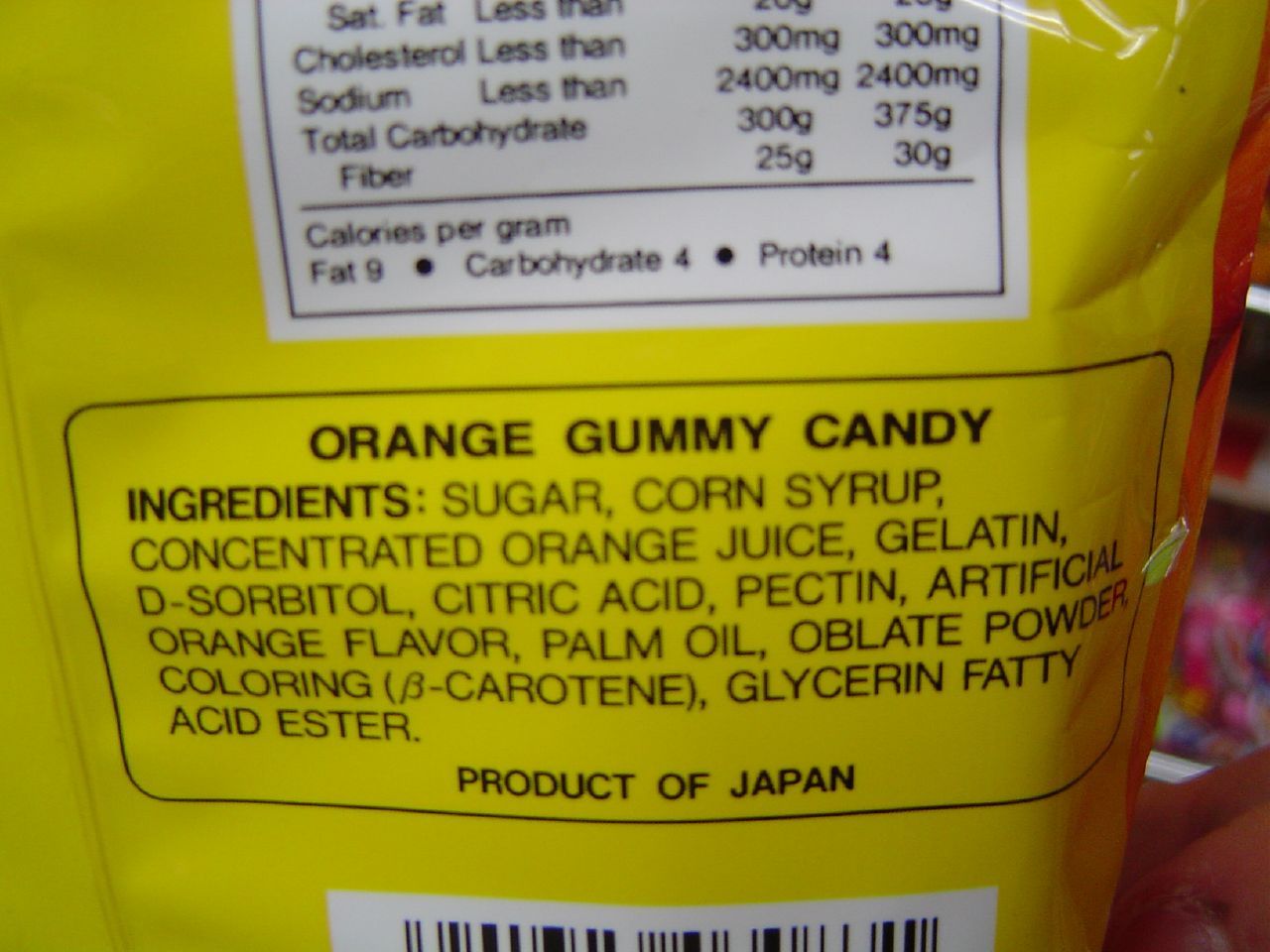This image is an extreme close-up photograph of a yellow plastic food package, specifically focusing on the nutrition facts and ingredient list. At the top of the package, partial nutritional information is visible in black text, indicating values for cholesterol (less than 300 mg), sodium (less than 2,400 mg), total carbohydrates (300 g), dietary fiber (25 g), and calorie values per gram for fat (9), carbohydrates (4), and protein (4).

Below the nutritional information, the package lists the ingredients for an orange gummy candy, printed in black font. The ingredients include sugar, corn syrup, concentrated orange juice, gelatin, D-sorbitol, citric acid, pectin, artificial orange flavor, palm oil, oblate powder, coloring (beta-carotene), glycerin, and fatty acid ester. The detailed close-up emphasizes the legibility and specificity of both the nutritional content and the ingredient list.